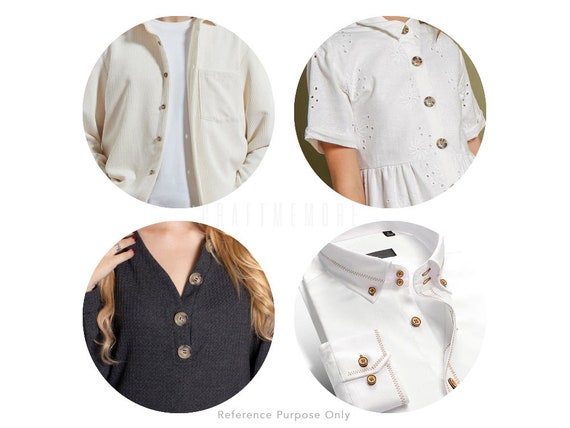This image features a unique collage of four circular photos, each showcasing different fashion pieces modeled by women. In the top left circle, a white T-shirt is layered beneath a long-sleeved beige dress shirt, resembling an outfit from Uniqlo. The top right circle depicts a girl in a white summer dress with four buttons down the center, reminiscent of a school or sailor outfit. The bottom left circle shows a woman in a dark, v-neck knit sweater with three large buttons, her long hair cascading down. The bottom right circle presents a white button-up shirt accented with brown buttons, a collar, and a pocket on the right side, neatly folded as though displayed in a store. The text "reference purpose only" appears in small gray print between the two rows of photos, suggesting this image is likely from retail or fashion advertising.